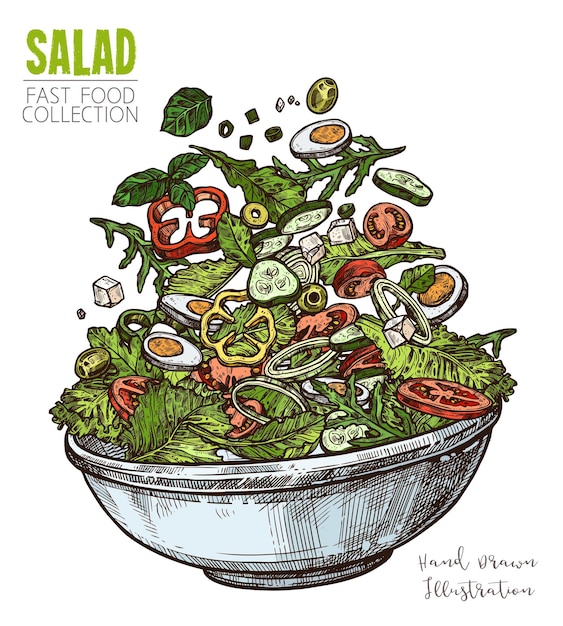A vibrant hand-drawn illustration features a cartoon salad, ingredients seemingly tossed up in the air above a bluish bowl with black lines. In the upper left corner, "SALAD" is prominently displayed in green capital letters, with "FAST FOOD COLLECTION" written just below in black lettering, separated by a black line. To the right of the bowl, in cursive black writing, it says "hand-drawn illustration." The salad includes a variety of colorful ingredients such as different types of lettuce (including green leaf), cucumbers, tomatoes, yellow bell peppers, onions, eggs with yolks, black olives, avocados, and perhaps some croutons. The white background makes this dynamic and colorful composition stand out, resembling an advertisement or a playful artistic representation of a tossed salad.